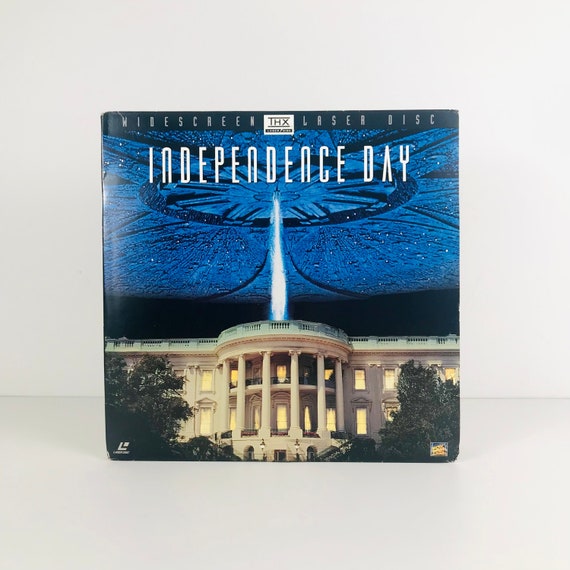This is a square photograph of a widescreen laser disc case for the 90s science fiction movie "Independence Day," which stars Will Smith and Jeff Goldblum. The case leans against a light gray wall, with a slightly different light gray surface beneath it acting as a counter or shelf. The cover prominently features the iconic promotional image of a massive alien saucer hovering over the White House, emitting a blue laser beam directly into the center of the rotunda. At the top of the cover, within a blue bar, white, all-caps sans-serif text reads, "WIDESCREEN LASER DISC," with a small THX logo between "WIDESCREEN" and "LASER." Below this, in bold white text, is the movie title, "INDEPENDENCE DAY." Additional logos, including the Laser Disc logo and the 20th Century Fox logo, are placed at the bottom left and bottom right corners. The image captures the vivid details, such as the yellow-lit windows of the Capitol and trees framing the scene.